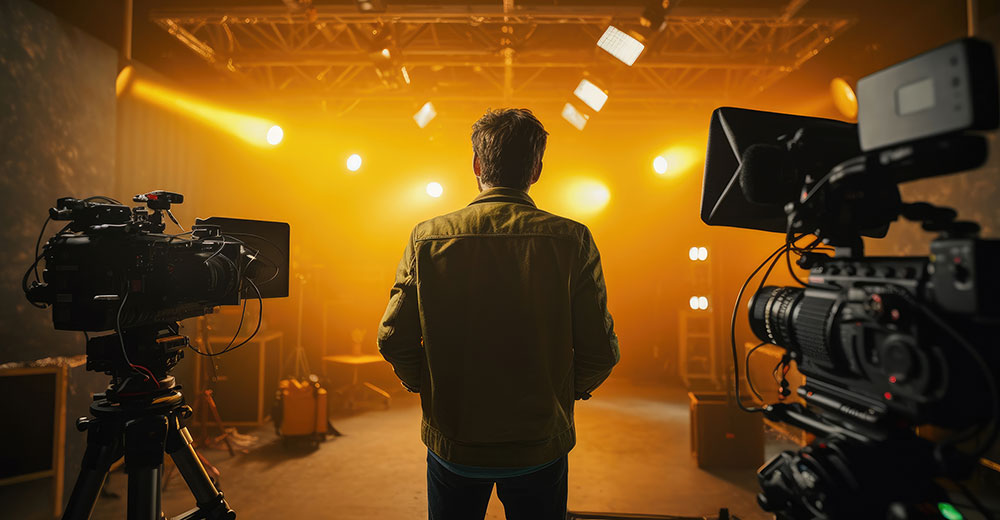The photograph depicts a studio set, potentially for a television show or movie, illuminated by bright, warm, yellowish-orange light. The space appears to be in the process of being decorated or set up, evidenced by the scattered items such as ladders, tables, and tools lying around. At the center of the image stands a man with his back to the viewer, perhaps an actor or crew member, wearing jeans, a blue shirt peeking out from underneath a tannish-green leather jacket, and sporting short brown hair with some facial hair. To his immediate left and right are sophisticated, large black cameras on tripods without any operators behind them. In the upper left corner, floodlights add to the intense illumination of the space, enhancing the orange hue that dominates the room. The overall composition suggests a behind-the-scenes glimpse of a studio set in preparation.